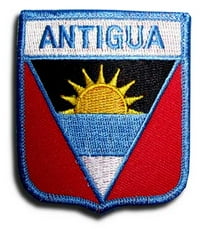This image depicts a detailed embroidered patch, likely intended for a uniform, representing the island nation of Antigua. The patch is centrally positioned, dominating the entire image, and crafted with vibrant colors including blue, white, black, yellow, and red. The patch is shield-shaped with a light blue braided border. Above, in a white rectangular section, the name "Antigua" is embroidered in light blue letters.

The central design of the patch features a black background with a yellow sun and its rays, which could be interpreted as either rising or setting. This image is flanked on both sides by red triangles. Below the sun, within a descending V-shape, are sections of blue and white symbolizing the sea and sandy beaches, reflecting Antigua’s island geography. The clear visibility of the embroidery and the shadow cast around the patch suggest that this is a photograph rather than a scan. The patch appears to be in three dimensions, showing the intricate woven details. This well-crafted insignia could be used for various purposes, such as for a collector, government official, or someone recently connected to Antigua.